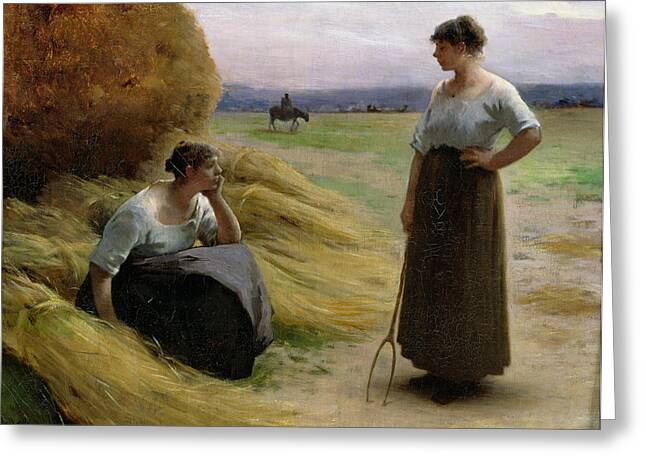This detailed oil painting depicts an outdoor pastoral scene featuring two women dressed in period attire. The woman on the left, seated thoughtfully on a bundle of hay, is dressed in a long, brownish-black skirt and a white blouse, with her hand resting pensively on her face. To her right stands another woman with similarly fair skin, also adorned in a long brown skirt and a white blouse, her hair neatly tied in a bun. She holds a two-pronged pitchfork and gazes at the seated woman. The standing woman's stance is confident, with one hand on her hip. Behind them, there is a slightly faded figure on horseback, possibly a man, adding depth to the scene. The background reveals a flat, grassy expanse transitioning into gentle, horizontal wisps of mountains under a sky filled with whitish-purplish clouds. The vibrant outdoor setting is also punctuated by an orange bush to the left and scattered patches of green grass.